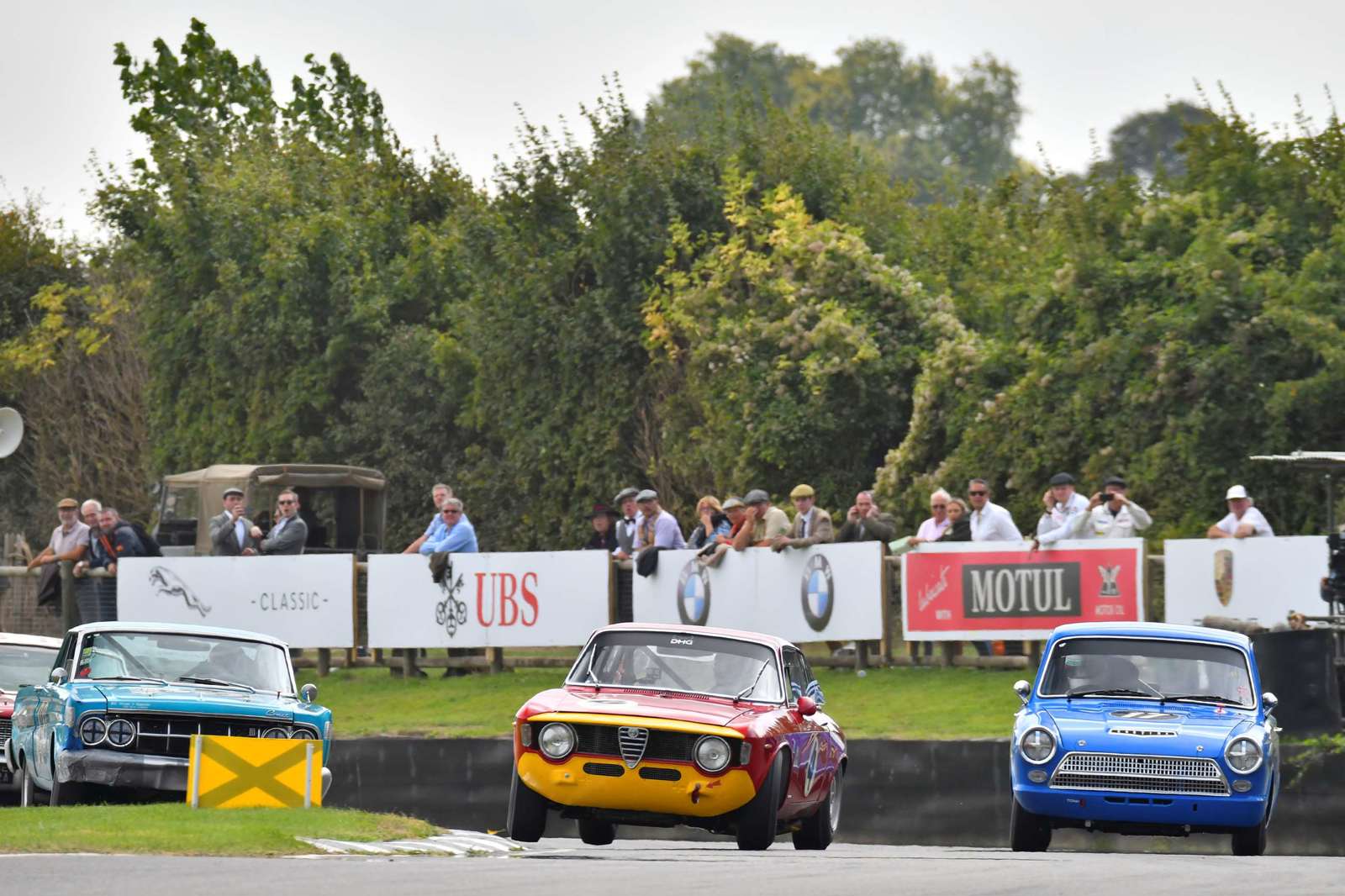This vibrant image captures the essence of a vintage stock car race on a classic racetrack. Dominating the forefront is a red car with a yellow front bumper, positioned almost head-on towards the viewer. To its left is a blue car, showcasing its front and right side. The red car features a noticeable blue stripe on its side. Nearby, a bright yellow flag with a large X is planted on a strip of green grass, suggesting a no-go zone.

Behind the action on the track, a diverse group of spectators stands on a grassy area, bordered by a brown wooden fence. The crowd, composed mostly of men dressed in an eclectic mix of attire—from modern casual wear to nostalgic olden-day outfits—gaze intently at the race. Some details include a man in a gray top hat, another in a tan suit with a tie, several wearing classic hats, and a bald man in a dark jacket on his phone, likely combating the noise.

Above the spectators, numerous advertisements are visible, including prominent BMW logos, a UBS sign in red and black, and a classic Mustang logo, adding a touch of commercial nostalgia. Beyond the human figures and the fence, a serene background of dense green trees frames the scene. The track itself is a slick black top, completing the picturesque atmosphere of this retro racing event.